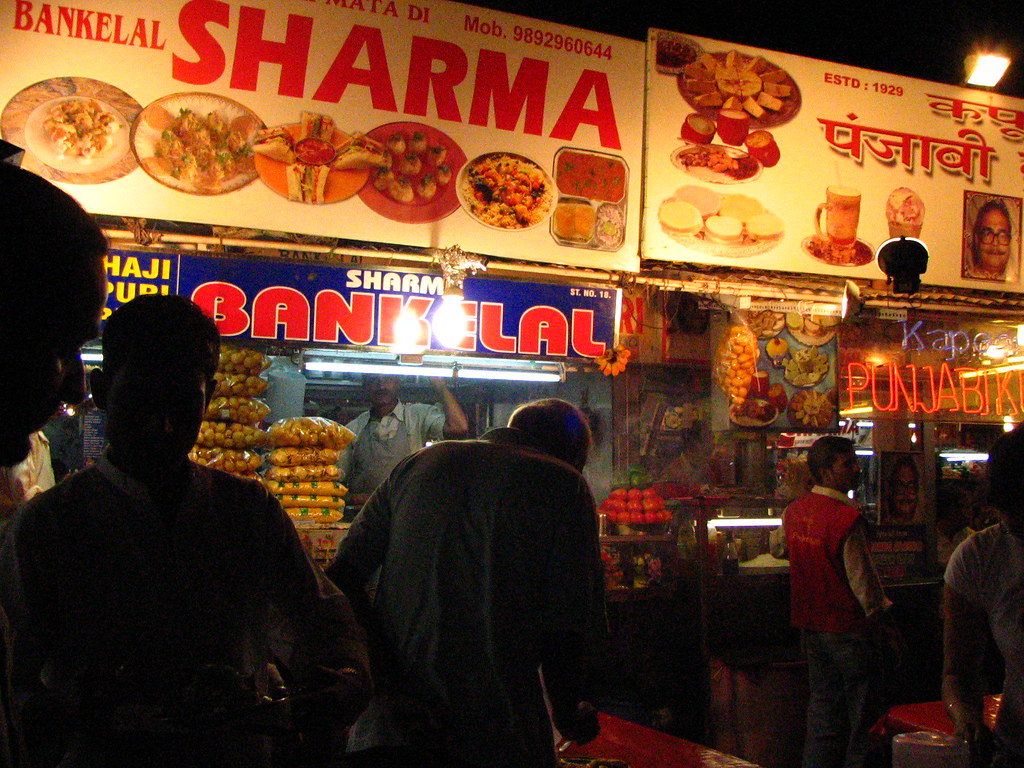The image portrays a bustling street food scene in India, captured during the evening or at night, indicated by the illuminated stalls and the darkened backdrop. Prominently featured is a food stall named "Bankilal Sharma," as highlighted by the large red text on a white background overhead. Below the main sign, there's a blue banner also displaying "Sharma Bankilal" in red text. This stall showcases various dishes such as sandwiches, pani puri, pav bhaji, and parathas, depicted on the signage. 

At the counter of the Bankilal Sharma stall, a man in an apron stands ready to take orders, illuminated by a small fluorescent light directly above him. Nearby, three people are noticeable on the left; two are engaged in conversation while the third seems poised to place an order.

To the right, another food stall is partially visible but somewhat obscured by the crowd. This stall features a sign with the words "Established 1921," and includes text in Hindi and English, mentioning "Kapoor Punjabi." This counter also displays various food items, with a light focusing on the sign and a picture of a person on it. The vibrant scene captures the lively atmosphere of Indian street food culture, with bright lights and a diverse gathering of people enjoying their evening at these popular food stalls.